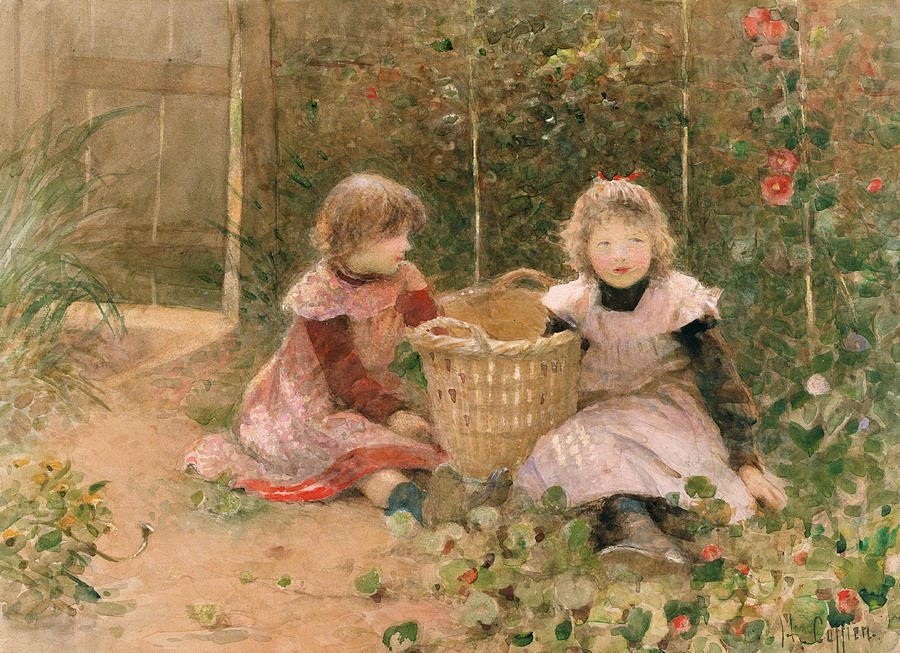This painting, signed by the artist H. Colleen in the bottom right corner, depicts two young girls sitting on the dirt in a lush garden surrounded by an array of green plants, vines, and vibrant flowers, including striking orange and possibly pinkish hues. The center of the painting features the two girls, immersed in their activity, with both of their arms nestled into a large wicker basket positioned between them. 

The girl on the right, appearing to be around five or six years old, has curly brown hair cut to about chin length. She gazes off into the distance, her expression steady towards the viewer. Her attire consists of a long brown shirt beneath a light pink ruffled dress, paired with brown shoes. 

The younger girl on the left, slightly turned to reveal a side view of her face, has dark chin-length hair and dons a bright red shirt beneath a frilly red and pink dress with an orange border. She, too, wears brown shoes as she leans towards the basket.

In the background, behind and surrounding the girls, are verdant plants and orange flowers. On the far left is a wooden slatted fence and gate, encircled by assorted weeds and more flowering plants, adding depth and a sense of enclosure to the garden scene. The girl's interaction with the basket amidst the serene, richly detailed garden environment is beautifully captured in this hand-painted acrylic artwork.